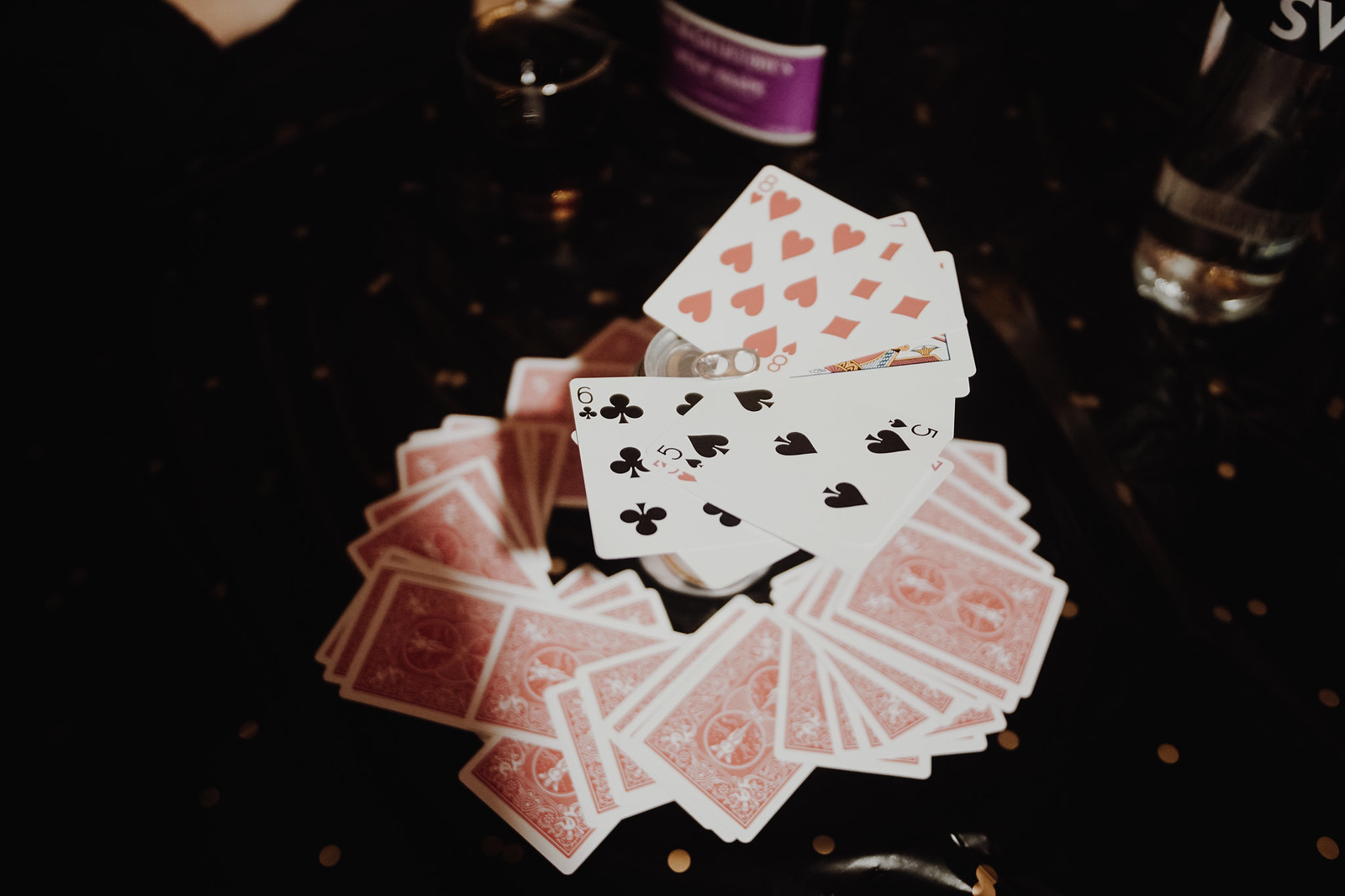A black table dotted with gold specks serves as the backdrop for a chaotic yet intriguing arrangement of playing cards. At the center, a collection of cards lies scattered, with most face down in a circular formation, possibly encircling an unseen object. Amid this array, approximately ten cards are face up, stacked and overlapping in a haphazard pile. Notable among them are the eight of hearts, seven of spades, six of clubs, five of spades, and three of hearts, along with an indistinct face card. The perimeter of the image is shrouded in darkness, revealing only partial glimpses of several glasses, the contents of which remain a mystery. The close-up focus and low lighting draw attention to the disheveled gathering of cards, evoking a sense of mystery and disarray.